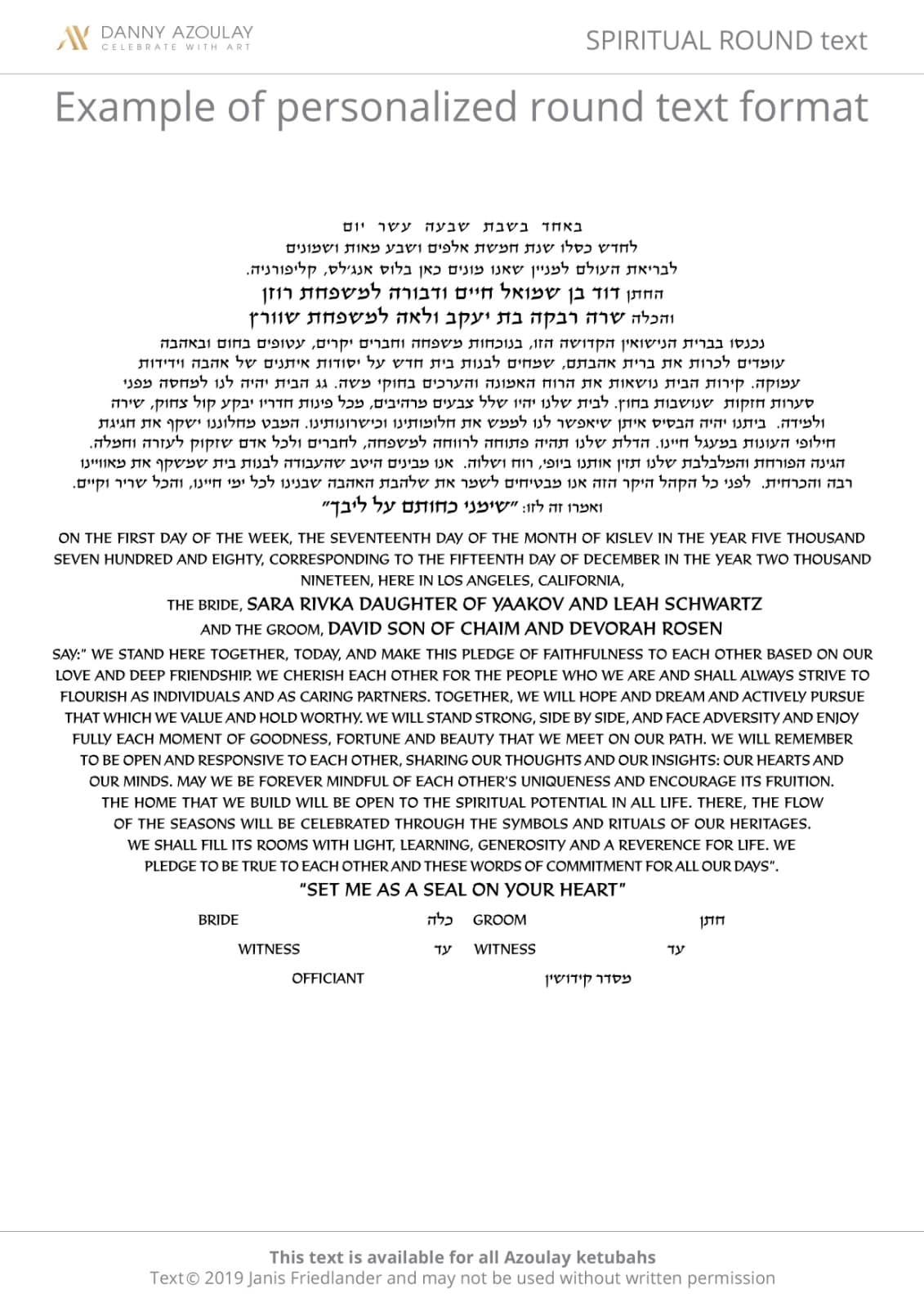This image showcases a personalized round text format, which is likely intended for use as a label on round containers like cans or jars. The content appears to be a wedding announcement, written in two languages, possibly Hebrew and English, with detailed decorative margins designed to fit a circular shape. At the top, the creator's name, Danny Azulay, is mentioned. The announcement details the marriage of the bride, Sarah Riva, daughter of Yakov and Leah Shorts, and the groom, David, son of Chaim and Deborah Rosen, which took place on the first day of the week, the seventh day of the month of Kislev in the year 5,780, corresponding to December 2019 in Los Angeles. The text conveys their vows, expressing their commitment, love, and aspirations for their shared life, emphasizing mutual respect, spiritual fulfillment, and an open, welcoming home. The phrase "Set me as a seal on your heart" is prominently featured at the bottom, encapsulating the spiritual significance of their union. The text is signed by both the groom and the bride.